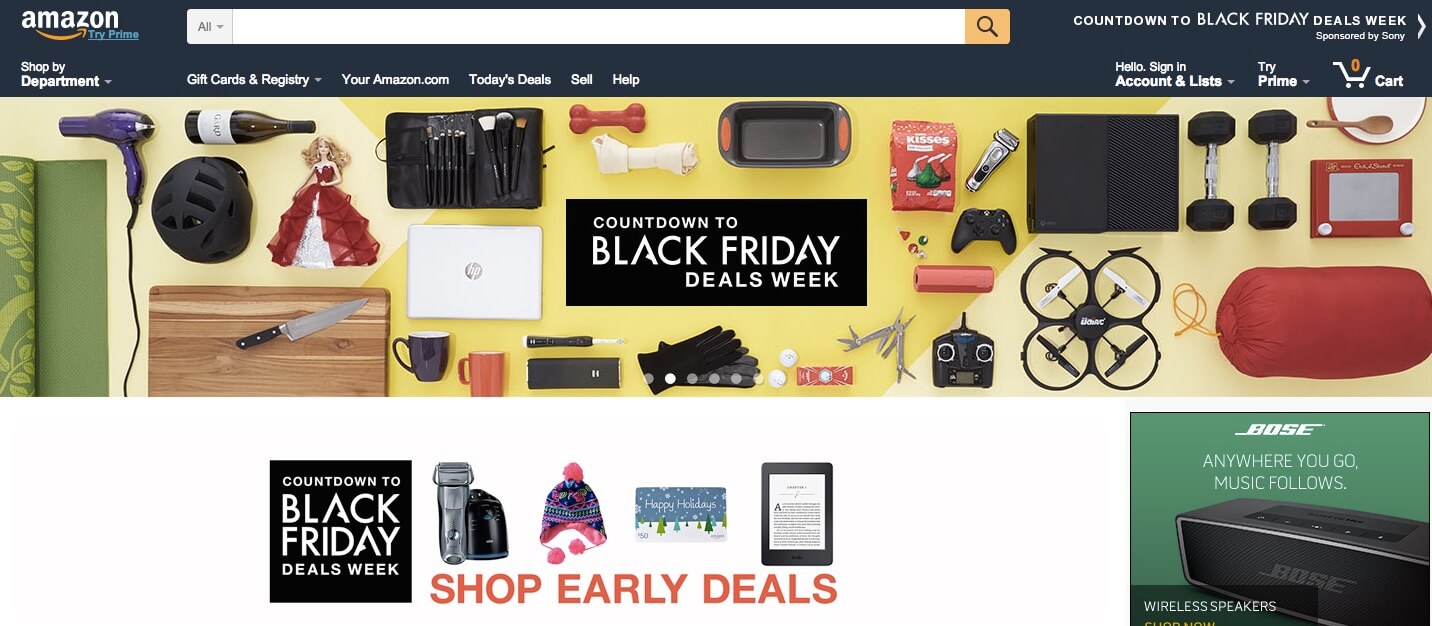This Amazon webpage screenshot offers a detailed view of various site elements and promotions. In the top-left corner, there is an "Amazon TryPrime" button, indicating that the user does not have a Prime membership. Centered in the top navigation bar is a search bar, while the top-right corner displays a "Countdown to Black Friday Deals Week" banner, sponsored by Sony.

Beneath this, on the left side, there's a "Shop by Department" dropdown menu followed by links for "Gift Cards & Registry," "Today's Deals," "Sell," and "Help." To the right of these links, there's a "Hello, Sign In Account & Lists" dropdown, a "TryPrime" dropdown menu, and a shopping cart icon showing zero items.

Below this navigation bar, the website showcases various product images including a purple hair dryer, a bottle of wine, a bicycle helmet, a knife and cutting board set, and a doll resembling one from the movie "Haunting Dolls 33 and a Third."